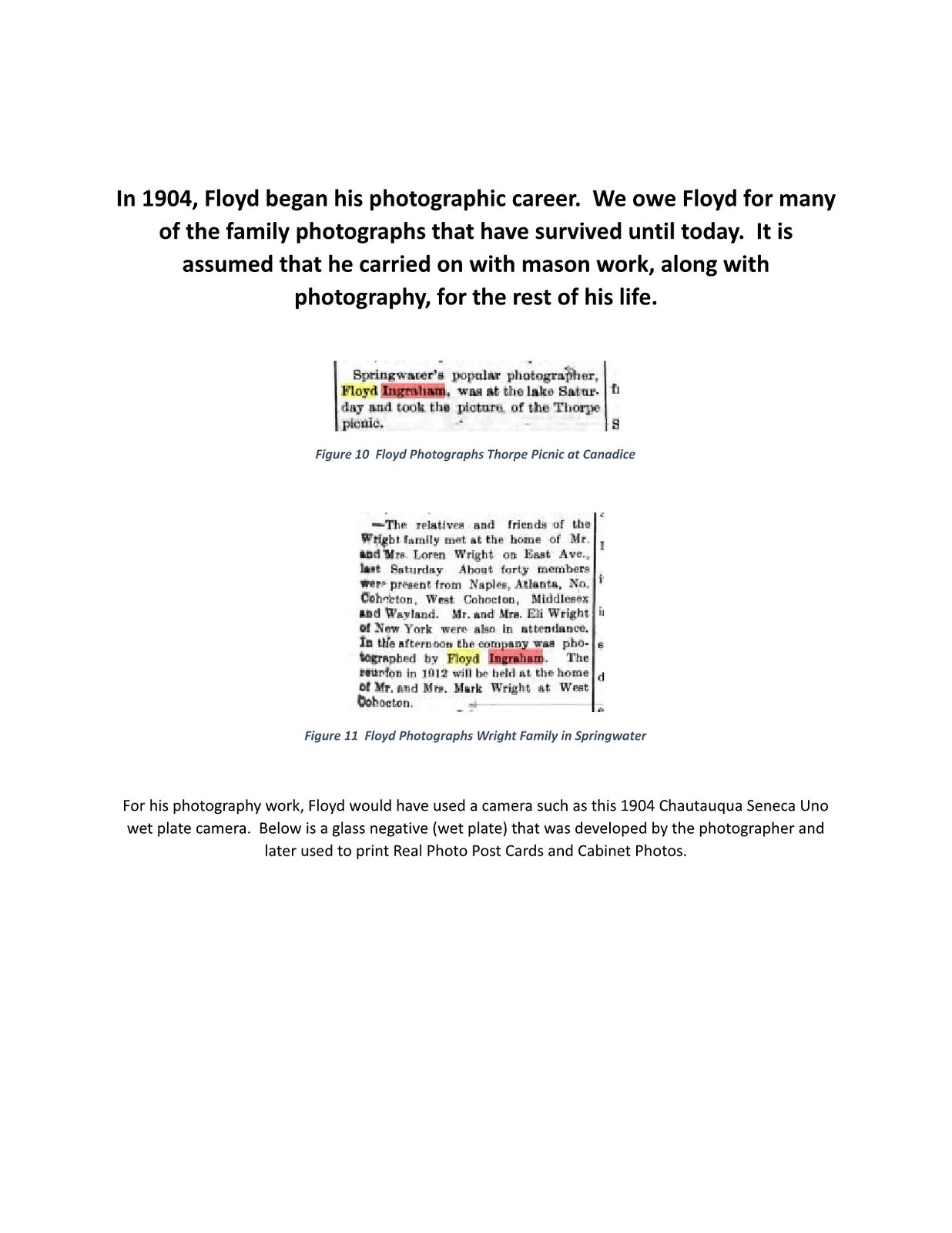This image features an old newspaper snippet prominently placed in the center. The article, highlighted with yellow and red accents, details the beginnings of Floyd Ingram's photographic career in 1904. It credits Floyd for the preservation of many family photographs still treasured today, and mentions his continued work as a mason. Specific events, like photographing the Thorpe family at Lake Saratoga and the Wright family in Springwater, are noted alongside figure labels 10 and 11. The text also describes the type of equipment Floyd would have used, specifically the 1904 Chattooga Seneca Uno wet plate camera. Below the main article, there's a depiction of a glass negative wet plate, used for creating real photo postcards and cabinet photos. The image itself has a predominantly black, white, gray, yellow, and orange color scheme, reinforcing the historical and archival nature of the content.